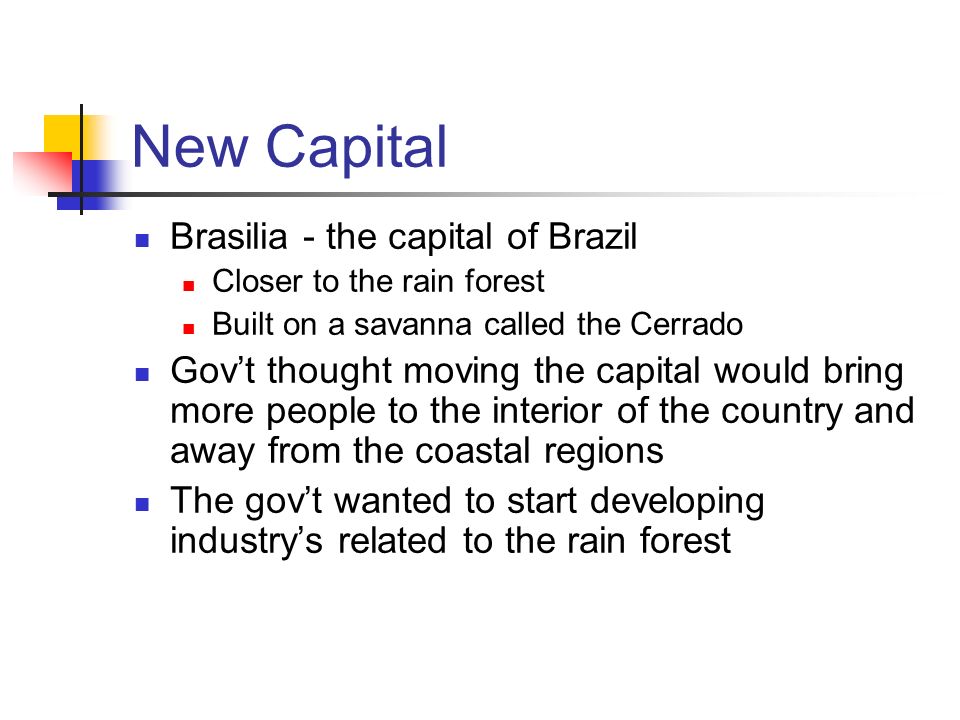The image displays a text-heavy page with a header and multiple points of detailed information. In the top left corner, the header reads "NEW CAPITAL" in blue capital letters. To the left of the "NEW CAPITAL" text, there's an icon consisting of three overlapping squares: a yellow square in the back, a red square in front on the left, and a blue square in the middle. A black vertical line runs through the center of the blue square, intersected by a horizontal line that extends to the right and gradually fades out.

Below the "NEW CAPITAL" header, there are three square bullet points, also in blue. Each bullet point contains black text. The first bullet point reads: "BRASILIA the capital of Brazil" and contains smaller red bullet points with the following information:
- "Closer to the rainforest, built on a savannah called Xerado."
- "Moving the capital will bring more people to the interior of the country and away from the coastal regions."
- "The government wanted to start developing industries related to the rainforest."

The text is written in black font, against a plain white background, making the information clear and easily readable.